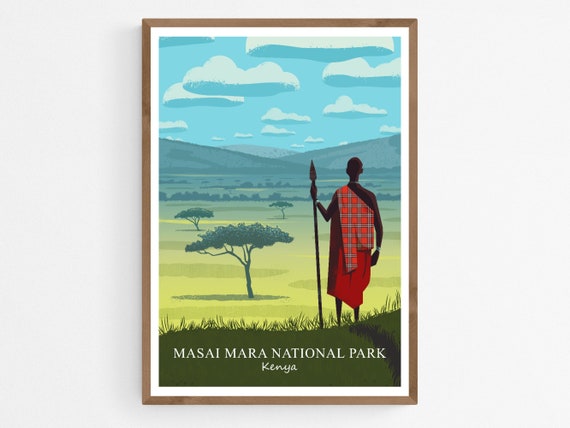A painting, framed with a light brown wood and a white mat on the inside, hangs on a white wall. The scene depicted is a vivid landscape of the Maasai Mara National Park in Kenya. In the foreground, an African man, adorned in a red cloak and a red tartan scarf draped over his shoulder, stands on an incline of green grass. He is holding a long spear in his left hand with the spearhead pointing upwards, almost reaching the sky, and his right arm rests by his side. The man, wearing traditional Maasai attire, turns his back to the viewer, gazing over the vast grassland. Scattered trees with unusual shapes are spread sporadically across the field, leading to blue mountains on the horizon. Above, a light blue sky is dotted with unique clouds that are flat on the bottom and medium blue and white on top. At the bottom of the painting, in white letters, it reads "Maasai Mara National Park, Kenya."